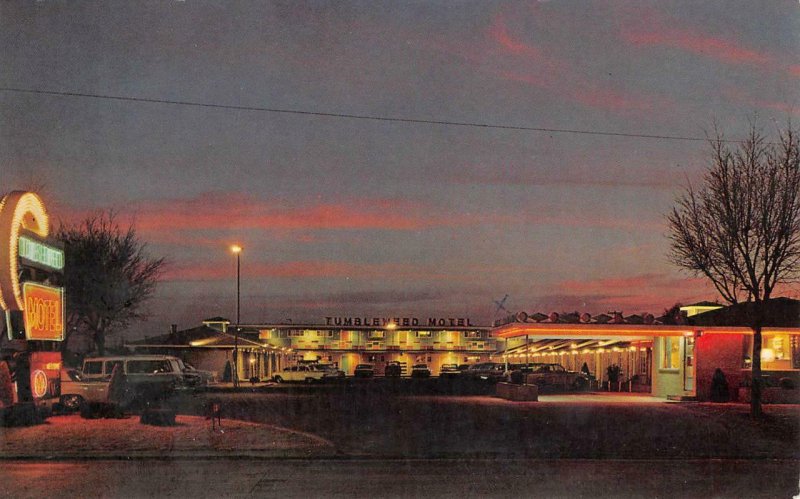The image captures a vintage or period photo, possibly from the 1960s, showcasing a dusk or sunset scene with a light blue sky and pink or golden clouds. In the foreground, there's a road running horizontally across the bottom of the picture. Just above this road lies a square parking area filled with vintage 60s cars. Dominating the center of the image is the two-story Tumbleweed Motel, its fluorescent lights brightly illuminating the scene. The motel building is rectangular and spans horizontally across the background. A neon sign on the left edge reads "Motel," but other text is obscured. There's a small tree on the right side of the image, and an electric line hangs midway through the scene. Although the lighting suggests it's quite dark, the motel is bathed in a mix of yellow, green, and orange lights. Scattered around are a few indistinct figures. The overall tone of the photo is hazy and atmospheric, with a nostalgic charm.